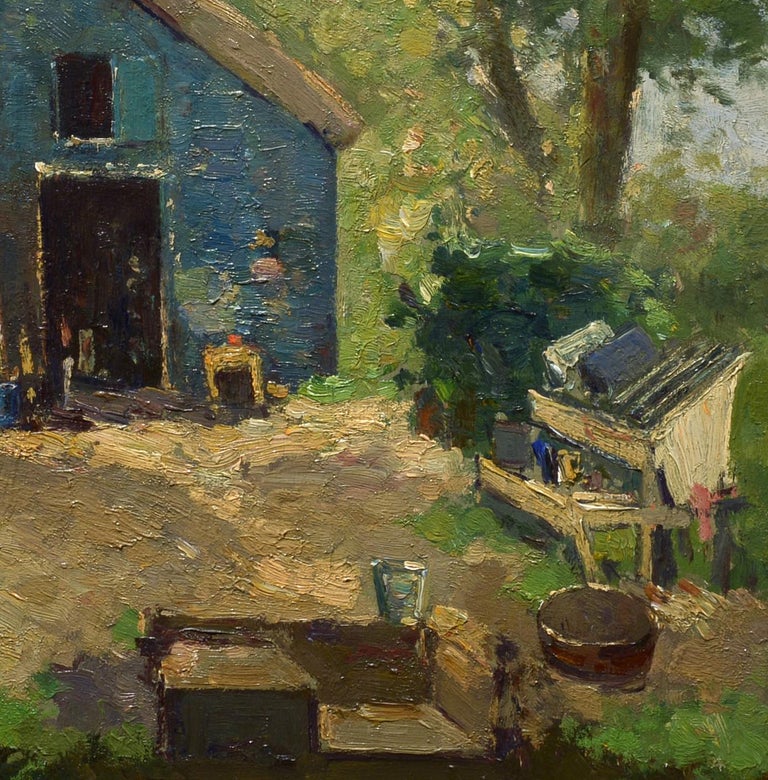This detailed oil painting depicts a large, dark blue barn set against a vibrant background of green, yellow, and cream hues. The barn features an open door and a small window at the top, both peering into shadows, adding a touch of mystery. Characteristic of the thick oil paint technique, the texture of the brush strokes is clearly visible, adding depth and dimension to the scene.

To the right of the barn, you can see tall trees with detailed green foliage, along with shrubbery and a bush near the ground. The scene at the bottom includes a dirt or hay-covered ground, with various work items scattered about. Notably, there is a rectangular wooden structure that appears to serve as a workbench or possibly an animal feeder, and nearby, a water bucket is situated next to a sitting area.

The painting's foreground also features what might be trays for paint or tools, adding to the atmosphere of a workspace. The background includes a glimpse of blue sky peeking through the tree foliage, completing the bucolic and rustic setting.